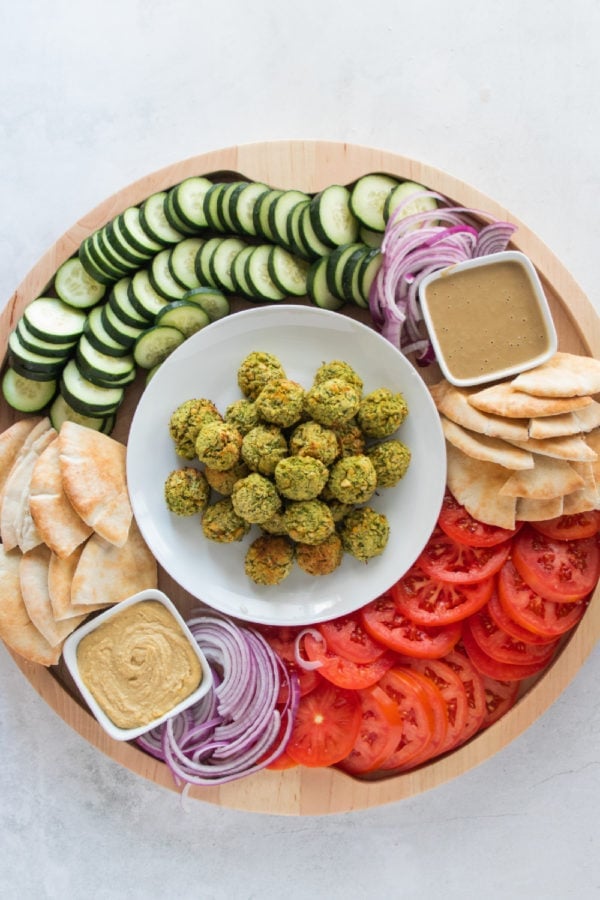The image features a wooden tray, resembling a charcuterie board, filled with an array of colorful food items primarily consisting of fresh vegetables and dips. In the center of the tray sits a white bowl containing approximately 10 to 15 small, round, green and brown falafel-like balls. Surrounding the bowl are various accompaniments. 

Towards the top section of the tray, there are numerous slices of fresh cucumber and slivers of red onions. In the lower right quadrant, bright red ripe tomato slices are neatly arranged. Scattered around the tray are pieces of pita or naan bread, and there are at least two distinct dips, one of which resembles hummus. The dips are positioned diagonally across from each other at roughly 1 o'clock and 7 o'clock or 2 and 8 positions.

The tray is set against a background that appears to be a white marble countertop, enhancing the vibrant colors of the food. The entire arrangement looks fresh and inviting, ready to be served at a gathering or party.